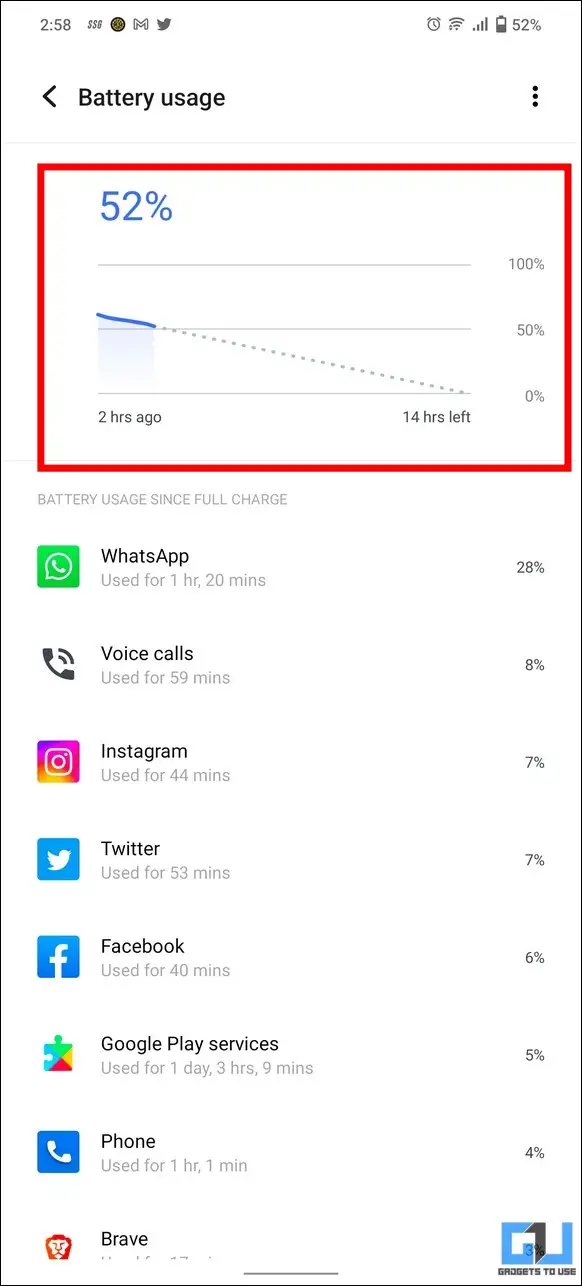Below is a cleaned-up and detailed caption based on the provided information:

---

The screenshot displays a smartphone's battery usage statistics. The status bar at the top shows various icons, including:
- A numeric indicator (258),
- Three currency symbols,
- A black circle,
- The letter "M",
- A bird icon (likely for Twitter),
- An alarm clock icon,
- Wi-Fi symbol with full signal bars,
- A data usage icon with full bars,
- Battery at 52% charge,
- Battery usage icon,
- Three vertical dots (more options),
- An arrow.

The main section of the image highlights the battery usage details, with a prominent red box emphasizing this information. The breakdown of battery consumption since the last full charge includes:
- WhatsApp: 120 minutes of usage, consuming 28% of the battery,
- Voice Calls: 59 minutes, using 8% of the battery,
- Instagram: 44 minutes, consuming 7%,
- Twitter: 53 minutes, also using 7%,
- Facebook: 40 minutes, consuming 6%,
- Google Play Services: continuous usage over 1 day, 3 hours and 9 minutes, consuming 5%,
- Phone app: 1 hour and 1 minute of usage, consuming 4%,
- Brave browser: an unspecified amount.

At the bottom center of the image, there is a horizontal line. In the bottom right-hand corner, the text "GU" appears with some black text beneath it, identifying the brand or specific feature related to the device.

The overall information provides insights into the battery consumption habits and app usage on the smartphone.